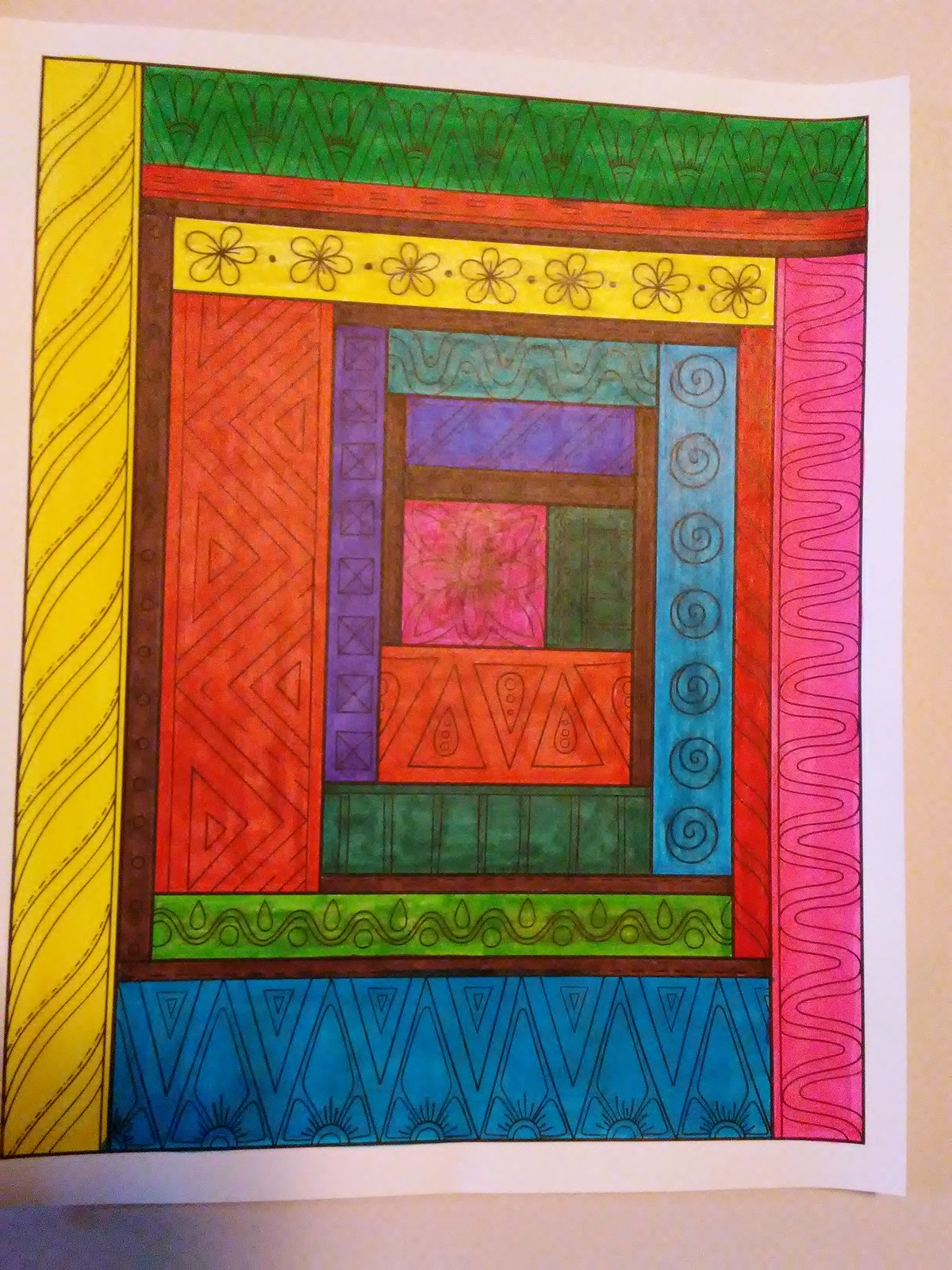The image is a top-down view of a coloring page positioned on a light pink table. The coloring page is bordered by a white frame, and its design is outlined in black ink. The composition features various geometric shapes, primarily rectangles, all meticulously colored with markers. 

On the left side of the coloring page, there is a long, thin vertical rectangle filled with horizontal lines. Above this section, a horizontal rectangle stretches across the page, adorned with diamond or triangular patterns in black outline. Below this rectangle is a thin, red horizontal strip that spans its entire bottom length.

Within the overall design, the page is segmented into multiple sections: horizontal and vertical rectangles, squares, and smaller rectangles, contributing to a complex and engaging pattern. The coloring is done with visible marker strokes, creating darker spots where the marker tips applied more pressure. The left vertical rectangle is colored yellow, while the right rectangle is pink. Other sections are filled with vibrant hues of red, green, yellow, and blue, adding a lively and dynamic feel to the artwork.